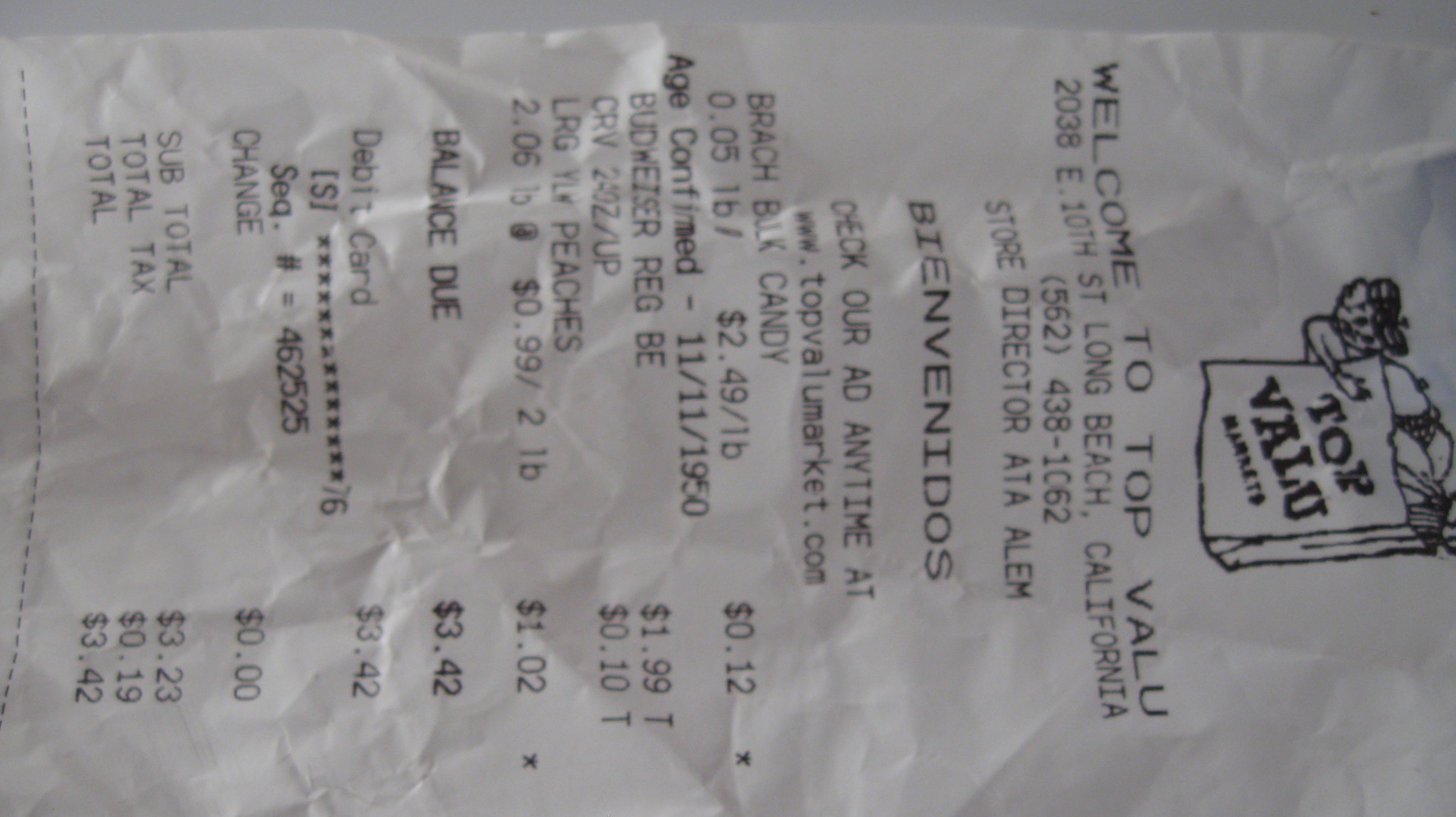This image features a crumpled receipt, presumably discarded and then retrieved by someone who realized they might need it. The receipt is placed horizontally on a countertop, with the top of the receipt oriented to the right side of the picture. 

The receipt is from "Top Value Markets," identified by its logo: a stick figure holding a large bag filled with produce and groceries. The store's address is 2038 East 10th Street, Long Beach, California, with the contact number 562-438-1062 and the store director listed as A. Alum. Additionally, the receipt includes a welcoming message in both English and Spanish: "Welcome to Top Value" and "Bienvenidos," respectively. 

It also promotes visiting their website at www.topvaluemarket.com. The listed purchases comprise candy, alcohol (with age confirmation), 7-Up, large yellow peaches, and various produce items. The total balance due on the receipt is $3.42, which was paid using a debit card. The receipt itself is typical of many grocery store receipts, albeit slightly crumpled, indicating it may have been casually discarded and then retrieved.